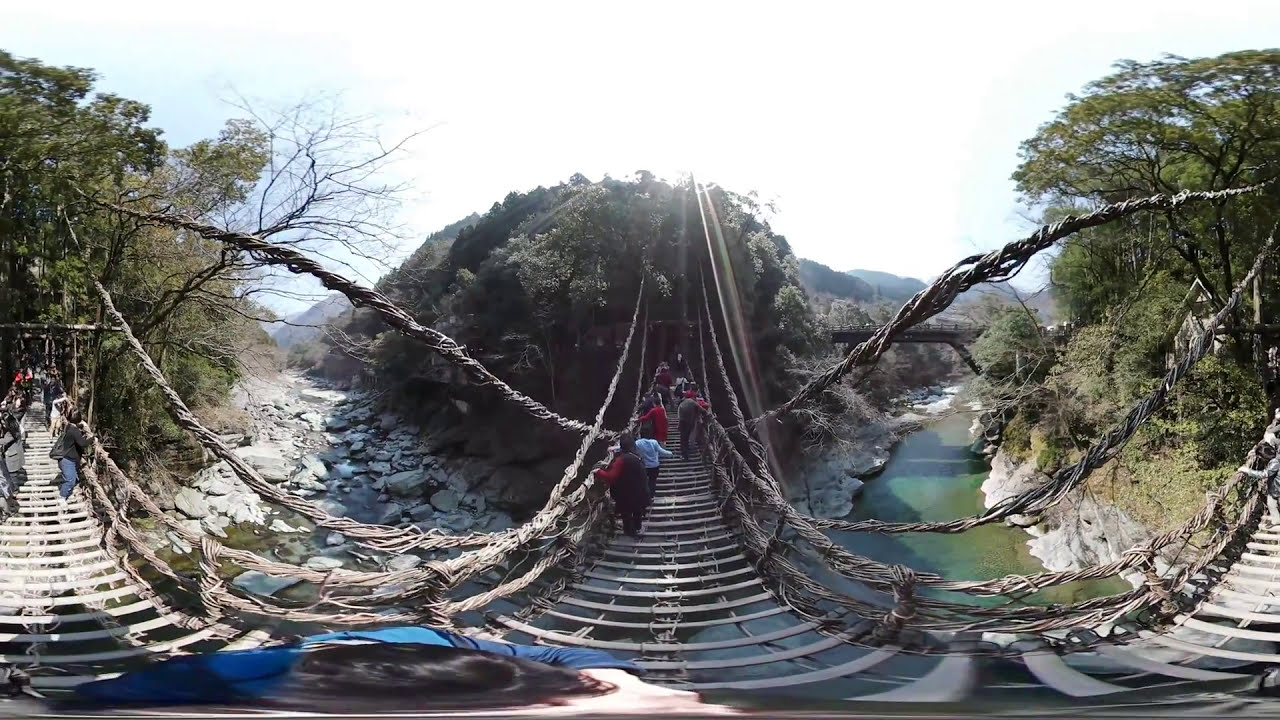In the image, we see three rustic, handmade wooden bridges, their sides beautifully entwined with tree roots and twigs, which serve as railings. They span different parts of a scenic outdoor area: one bridge is to the right, another to the left, and one in the middle. The middle bridge stretches across a large, greenish river with sandy-colored rocks and boulders, while the left bridge arches over a smaller stream. The right bridge is distantly elevated, sitting approximately 40-50 feet high in the air, and there's another more modern bridge visible in the panoramic background. 

People are crossing these bridges, especially the middle one, where a cluster of individuals in red and white jackets can be seen. They are holding onto the railings, looking out towards the river and the lush forest behind. On the left bridge, more casually dressed individuals in red jackets also gaze at the flowing water below. The scene is bright and inviting, set against a sky with a hint of blue and punctuated by the presence of hills and possibly mountains in the distant background. The entire setting is lively with a touch of natural wilderness, captured in a slightly warped panoramic view, adding a sense of depth and immersion to the image.